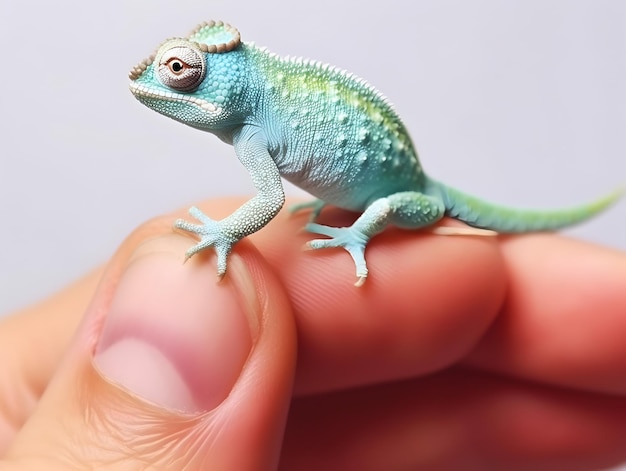In this highly detailed close-up image, a Caucasian left hand is featured, holding an incredibly tiny, newborn chameleon. The background is a medium gray, which accentuates the vivid colors of both the hand and the chameleon. The hand is positioned such that the thumb, index, and middle fingers occupy most of the bottom half of the image. The thumb, prominently displayed in the lower left quadrant, reveals intricate skin textures and miniature wrinkles due to the extreme zoom level.

Perched precariously between the thumb and the index finger is the small chameleon, no larger than the top knuckle of an average finger. This mint green reptile, with a seafoam hue, rests with its front paw delicately gripping the top of the thumb. The chameleon features a lighter green stripe running along its back and tail. Additional detailing includes a series of brown dots lining its body from its mouth, around the back of its head, and down the other side. It also sports a tan stripe over its mouth area, and its eye is a matching tan color. The tiny chameleon’s claws, appearing as a light khaki shade, cling faintly to the thumb, emphasizing its diminutive size. Overall, the photograph captures the delicate beauty and intricate details of both the hand and the tiny reptilian creature.